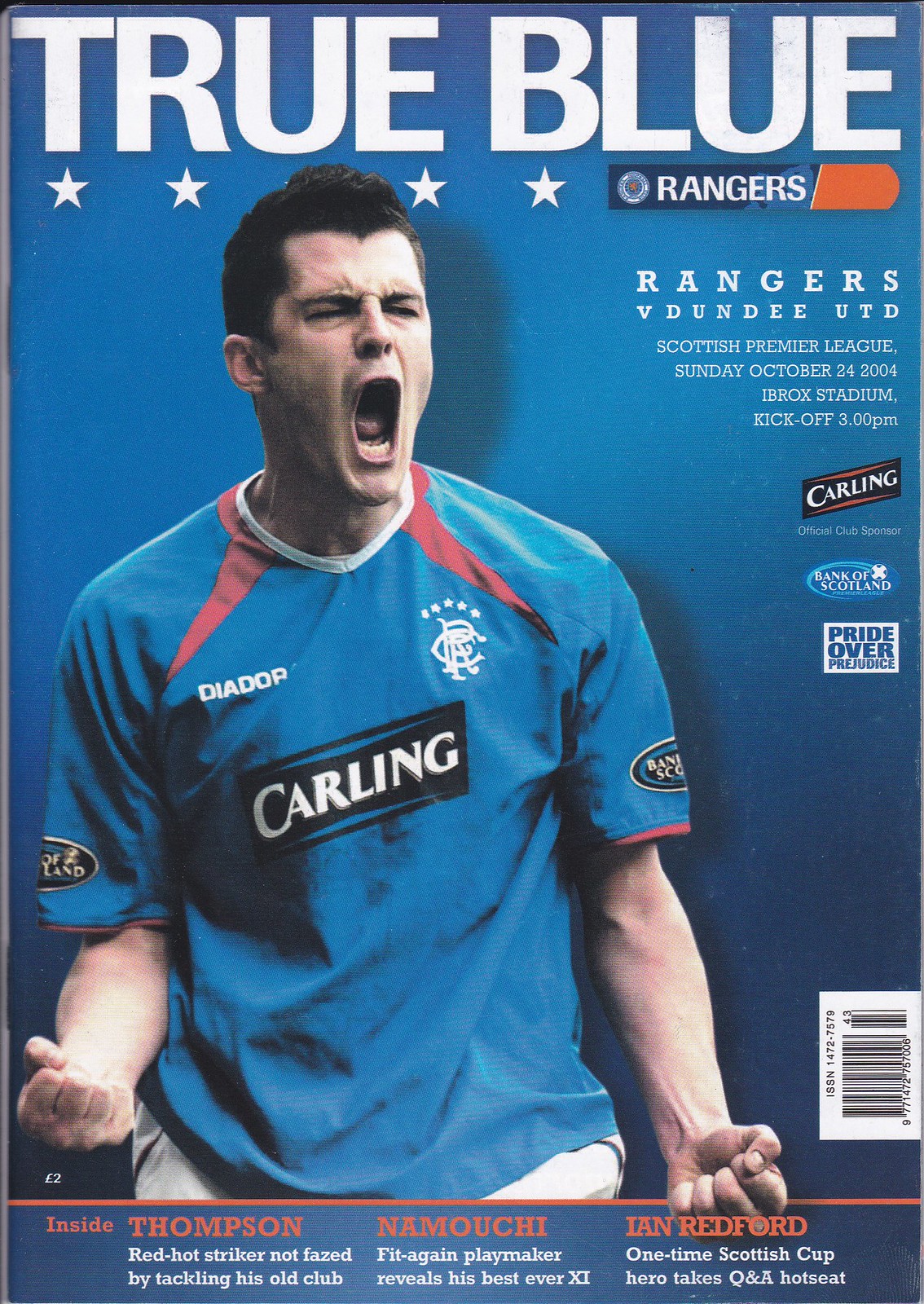The cover of this soccer magazine features an image of an electrified player, dressed in a blue uniform with a distinctive white collar and red stripe, emblazoned with the sponsor 'Carling' in white lettering set against a black rectangle with blue lines. The player, appearing to be part of the Rangers team, has short dark hair and is captured in a moment of intense excitement, with both fists clenched and his mouth open in a triumphant yell. This dynamic pose takes up most of the cover, set against an all-blue background.

At the top of the magazine, the title "True Blue" is prominently displayed in bold white text, beneath which a row of five stars appears - though only four are fully visible as the player's head obscures part of one. Below this, the heading reads "Rangers vs. Dundee United, Scottish Premier League, Sunday, October 24, 2004, Ibrox Stadium, kickoff, 3 o'clock p.m."

Various sponsor logos are visible, including "Carling" again along the sleeve and near the bottom right of the cover where a barcode also appears. Across the bottom, in vibrant orange text, the magazine highlights featured content: "Inside: Thompson, Namouchi, and Ian Redford," indicating exclusive insights or articles on these players. The player's blue uniform also features a club emblem on the left upper shoulder, enhancing the sense of team pride and identity. The overall design of the magazine cover, with its rich blue hues and compelling imagery, effectively captures the excitement and fervor of the match day.